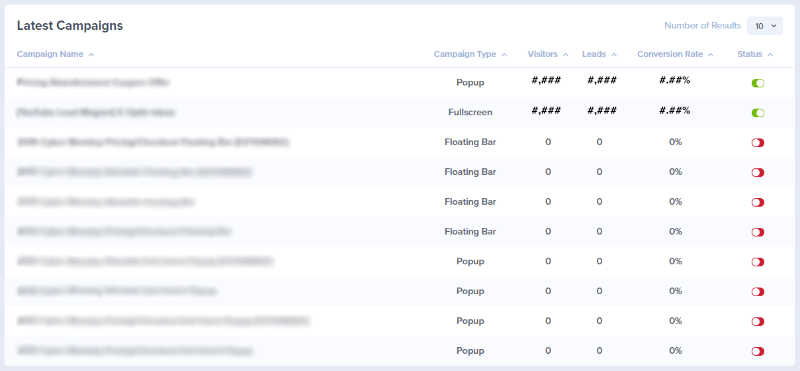The image depicts a large, rectangular interface longer in width than height, titled "Latest Campaigns" at the top. Below this title, a section labeled "Campaign Name" lists ten campaign names, which have been blurred out to maintain privacy. Adjacent columns provide additional campaign details, including "Campaign Type," "Number of Visitors," "Leads," "Conversion Rate," and "Status."

In the "Campaign Type" column, the first campaign is categorized as "Pop-up," followed sequentially by "Full Screen," a series of "Floating Bar" entries, and concluding with more "Pop-ups." The "Number of Visitors" column displays hashtags in the top two rows, while the rest are marked as zero. Similarly, the "Leads" column follows the same pattern.

Under "Conversion Rate," the top two rows contain a mix of hashtags or percentages, but the remaining entries state "0%." The "Status" column indicates that two campaigns are active, shown in green, while the others are inactive.